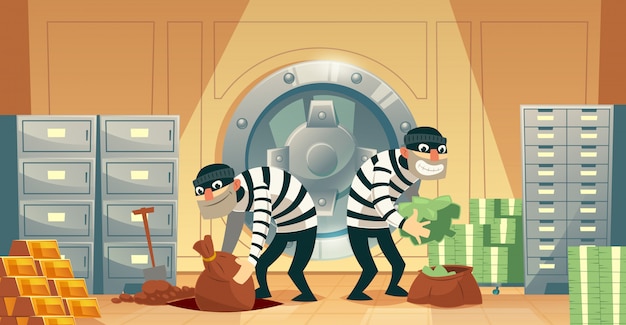In this detailed cartoon illustration, two bank robbers are depicted in the midst of a heist inside a bank vault. Both burglars are clad in classic black and white striped shirts, black pants, black beanies, and have black bandanas over their eyes, with noticeable five o’clock shadows adding to their criminal appearance. The guy on the right is busily loading stacks of cash into a brown satchel, while his accomplice on the left is bent over, reaching down to place a tied-off, full brown bag of money into a hole they've dug in the floor. The background showcases beige walls with a circular silver knob marking the vault entrance, flanked by safe deposit boxes. Notably, there are stacks of gold bars neatly piled in the lower left corner and bundles of cash in the lower right, emphasizing the hefty loot they've amassed. This scene likely represents a moment of tense, illicit activity with an escape plan already in motion.